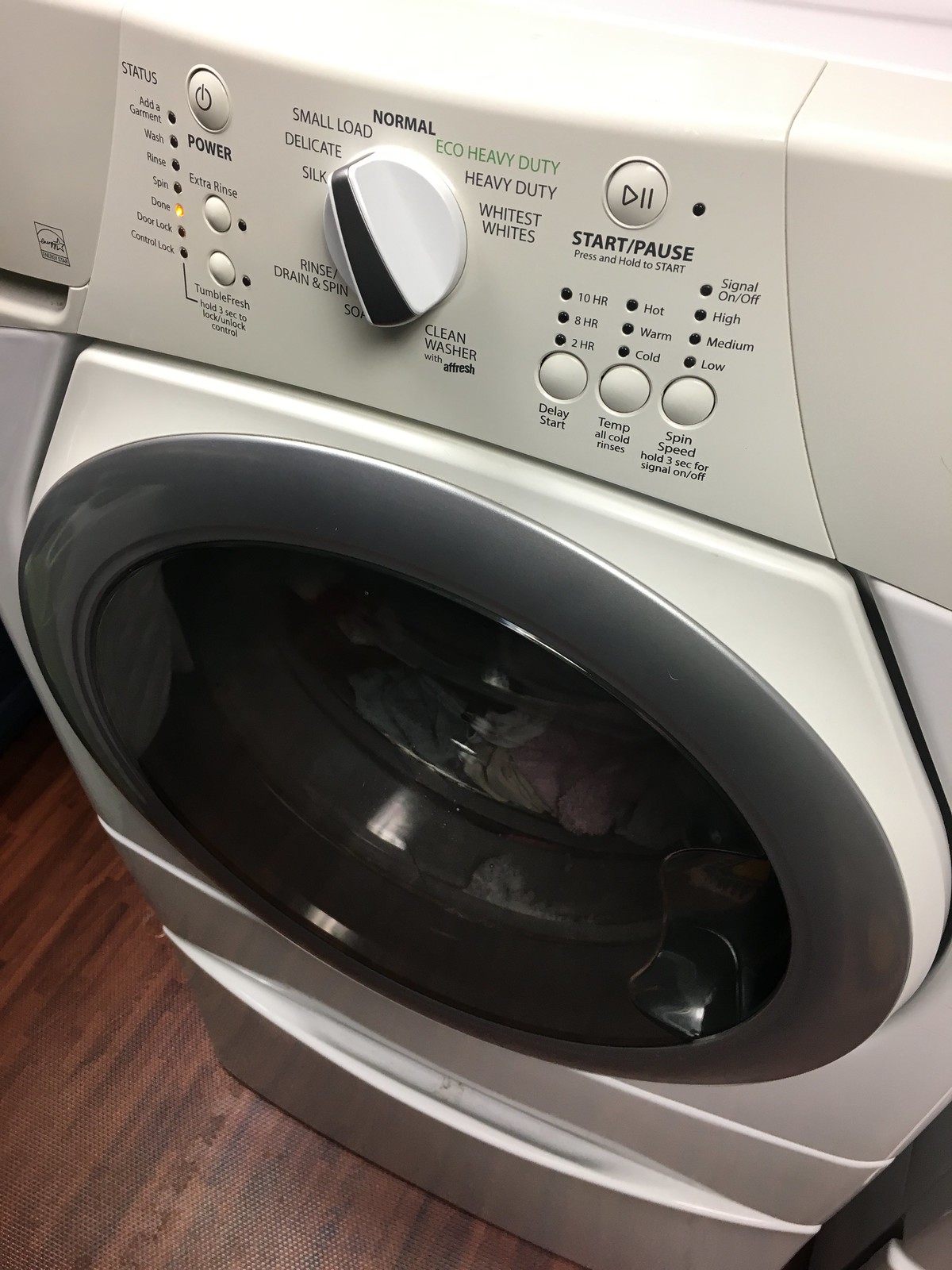This image is a close-up, downward angled photograph of a front-loading, Energy Star-rated washing machine standing on a wood grain puzzle mat floor. The washer itself is a cream color with a dark gray door featuring a circular glass window, which is closed. The control panel at the top center includes a rotary switch for selecting wash settings, ranging from Normal, Small Load, Delicate, Silk, Eco-Heavy Duty, Heavy Duty, to Whitest Whites. To the left of the dial, there is a main power button and two additional white buttons likely for extra rinse or other functions. On the right side of the panel, there is a Start-Pause button, along with various buttons and an LED display for setting the water temperature, spin speed, delay start, and timer functions. The washer has a drawer at the bottom, possibly for lint collection or storage.